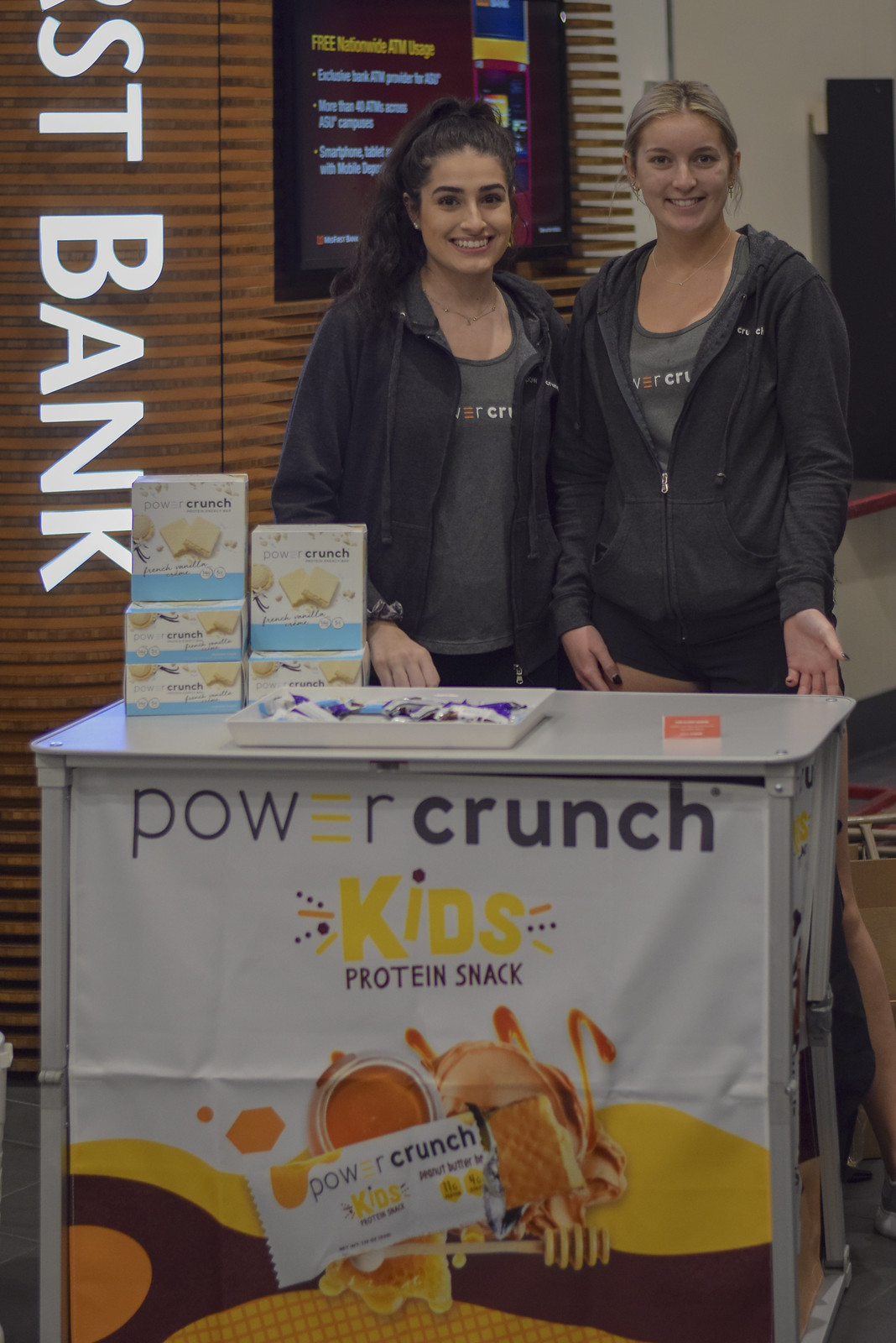In this indoor photograph taken at a First Bank, two young teenage girls stand behind a waist-high white podium promoting Power Crunch Kids Protein Snack. The girl on the left has long black hair styled in a ponytail and wears a black zip-up hoodie over a tan tank top, paired with a friendly smile. The girl on the right, slightly taller with blonde hair also pulled back, is dressed similarly. They're positioned in front of a striped curtain with wooden paneling and a television screen displaying bank information, including the bank’s logo and services like free nationwide ATM usage. The podium in front of the girls features a banner showing the Power Crunch Kids Protein Snack logo and an image of the wafer-style snack, which appears to be honey and peanut butter flavored. On the podium, there are several boxes of the product along with a tray of sample bars neatly arranged for distribution. The setting is illuminated by fluorescent lighting, and both girls smile warmly at the camera.